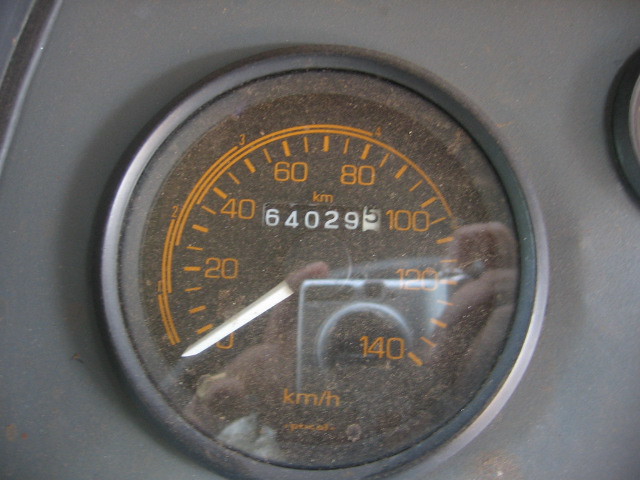The photograph displays a car's dashboard against a gray background. The dashboard appears to be made of vinyl. In the upper left corner, there is a darker gray strip running diagonally. At the center of the image is a circular speedometer encased in plastic, featuring a dark gray frame and a protective glass cover. The reflection of the camera and the photographer’s hand is visible on the glass. The speedometer displays speeds in kilometers per hour, marked with the numbers 0, 20, 40, 60, 80, 100, 120, and 140 in orange, arranged in a semicircle. The odometer reads 64,029.5 kilometers. In the upper right corner, there is a partial view of another gauge, though its specific function is indiscernible.